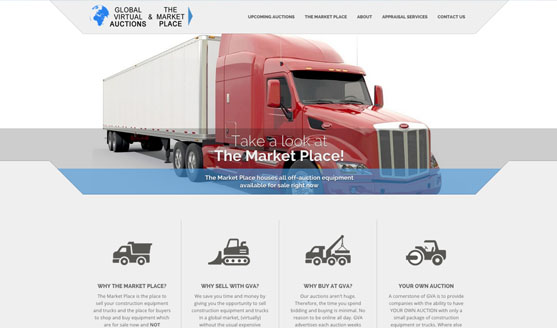Here is the cleaned-up and detailed caption for the image described:

---

The image depicts a web page displayed on a desktop computer screen. At the top of the screen, there is a grayed-out header containing black text that reads, "Global Virtual Auctions and Their Marketplace." Just below this header, set against a white background, is a large truck prominently featured. The truck has a red cabin and a white body, indicating it is a container truck. Written in white text on the front and partially along the side of the red cabin is the phrase, "Take a Look at the Marketplace." Beneath the truck image is a blue framed section with additional text in small white print, providing more details. At the very bottom of the page, there is a light gray footer area displaying four icons from left to right: a truck icon, and next to it, an icon of large construction equipment.

---